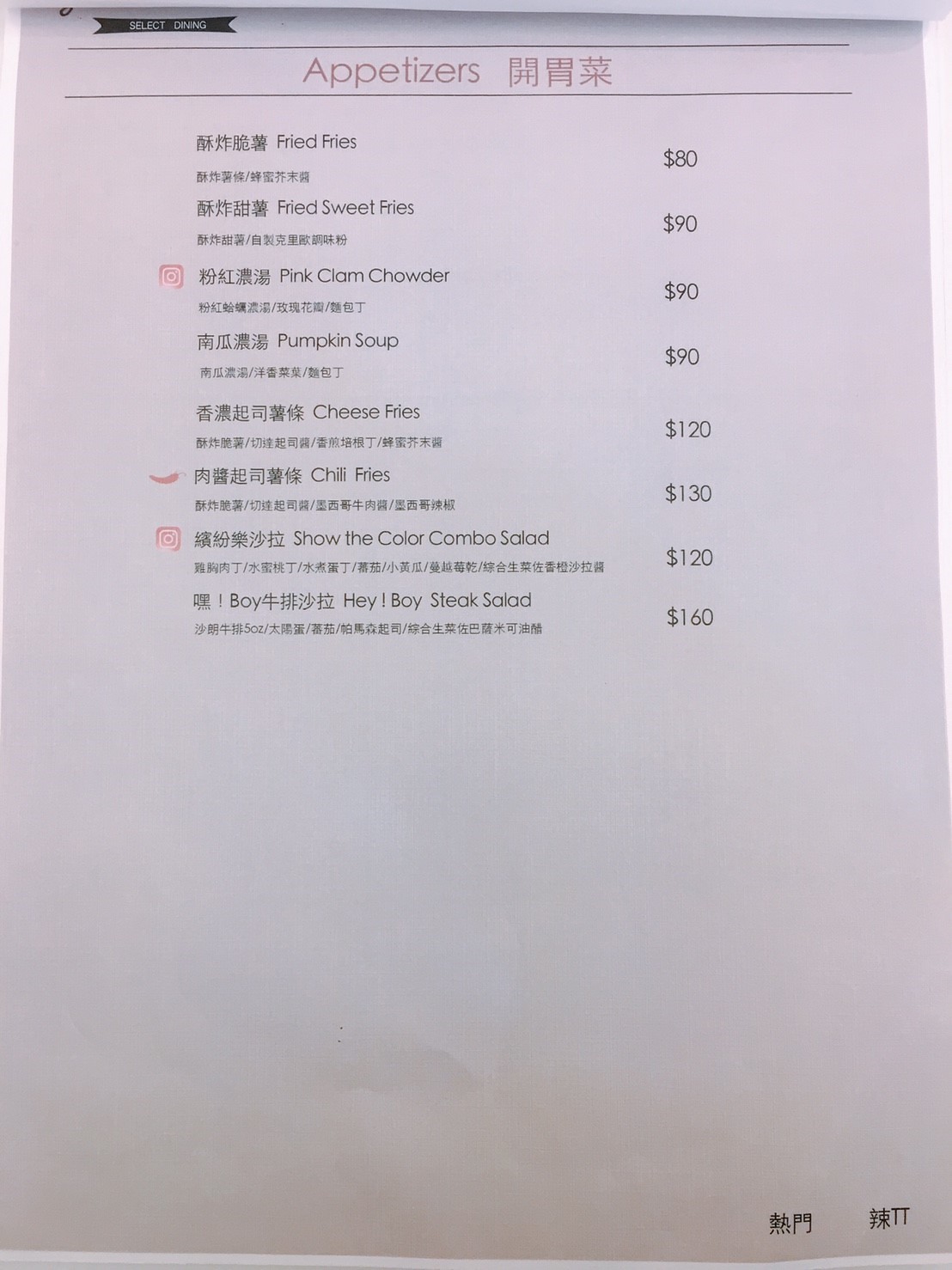The image displays a white menu with the word "Appetizers" prominently printed at the top in red font. Adjacent to this is the Japanese or Chinese translation of "Appetizers." Below, the menu lists various items along with their translations in Japanese, English, and possibly Chinese. Each item is followed by its price, listed to the right.

Readably, the items include:
- Fried Fries - $80
- Fried Sweet Fries - $90
- Pink Clam Chowder - $90
- Pumpkin Soup - $90
- Cheese Fries - $120
- Chili Fries - $130
- Show the Color Combo Salad - $120
- Hey Boy Steak Salad - $160

Some items feature small icons beside their names, adding visual cues:
- Pink Clam Chowder features an Instagram icon.
- Chili Fries is marked with a red chili icon.
- Show the Color Combo Salad also includes an Instagram icon.

The bottom right corner of the menu contains additional text in Japanese or Chinese. At the top left, the words "Select Dining" are displayed.